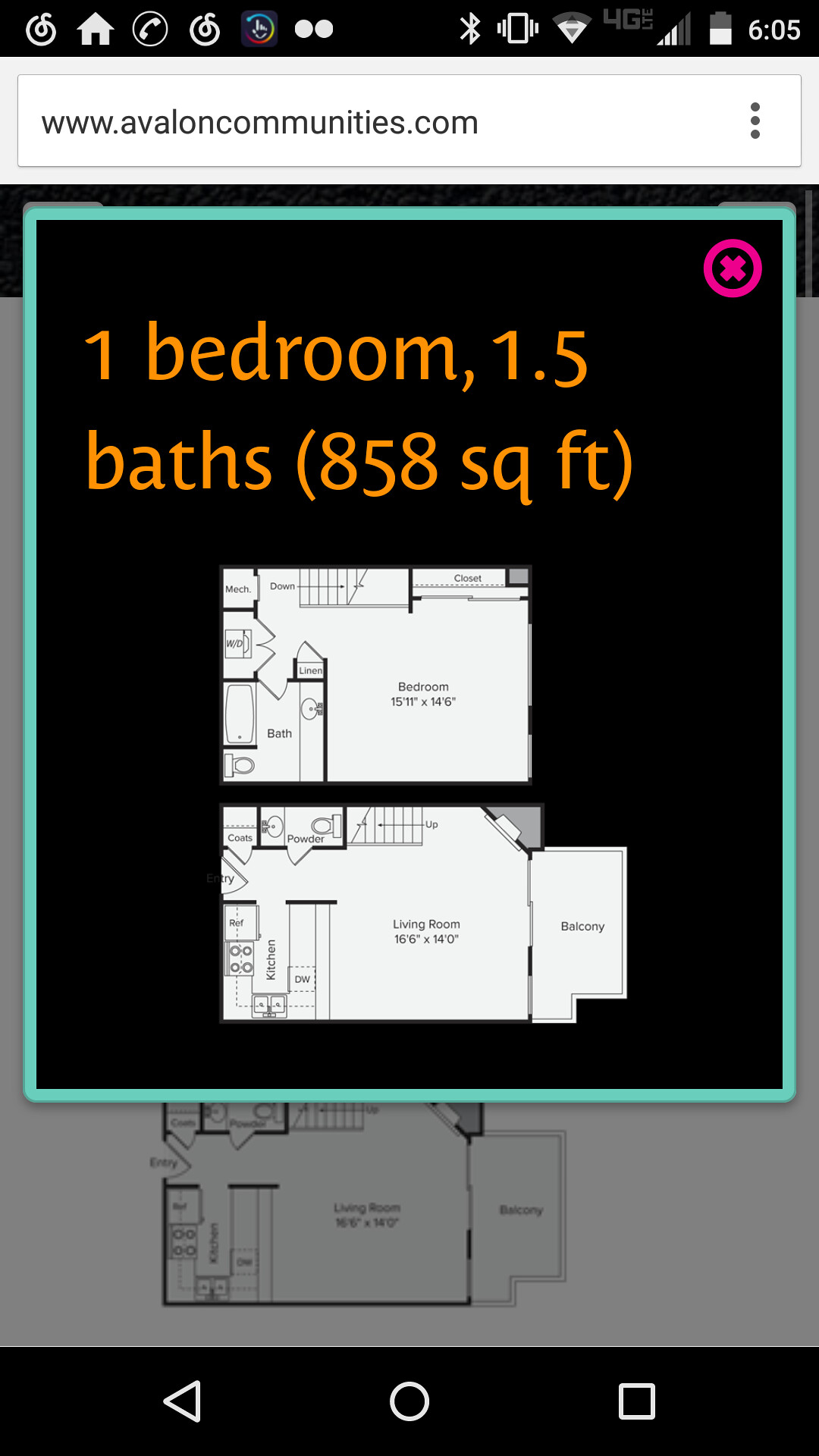A detailed screenshot of a floor plan for a home displayed on a person's phone from the website www.avaloncommunities.com. The top of the screen features typical phone icons against a black bar, including a home icon and the WhatsApp logo, along with the time 6:05 visible in the top right corner.

The primary image shows a floor plan set against a black background with a vibrant blue border. In the top right corner is a magenta circle containing a magenta “X.” The text “One Bedroom, 1.5 Baths (858 square feet)” is displayed in orange beneath the magenta circle.

The floor plan is divided into two main sections:

1. **Upper Section (Bedroom)**
   - Shows a detailed layout of the bedroom.
   - Features a bath positioned in the corner and a closet in the top right section.
   - Includes a staircase descending from the bedroom area.

2. **Lower Section (Living Room)**
   - Dimensions are labeled as 16 feet 6 inches by 14 feet.
   - Contains a small bathroom in the top left corner.
   - The kitchen is located in the bottom left corner.
   - There is also a balcony adjacent to the living room area.

In the background, a smaller white screen mirrors the same floor plan layout, providing an additional view of the home’s layout.